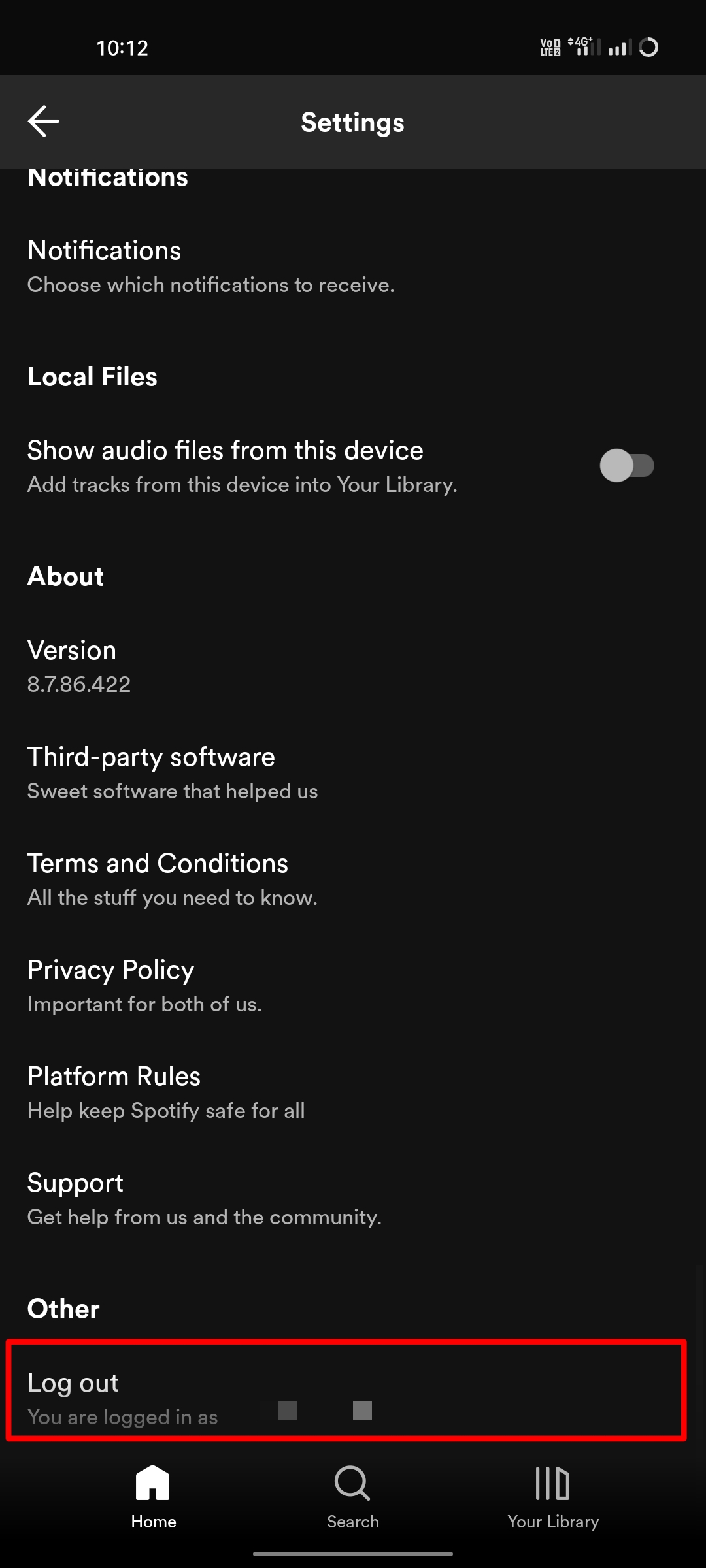A screenshot captured from a cell phone shows the device's settings menu against a black background. The majority of the text is in white, with some areas appearing slightly grayish. At the top, there is a back button labelled 'Settings,' followed by a 'Notifications' section with the prompt 'Choose which notifications to receive.' Below that, there is an option for 'Local Files' with a description that reads 'Show audio files from this device,' which is currently turned off, as indicated by the slider positioned to the right. Another line below states 'Add tracks from this device into your library.'

Further down, the 'About' section lists various items including 'Version,' 'Third Party Software,' 'Terms and Conditions,' 'Privacy Policy,' 'Platform Rules,' and 'Support,' followed by an 'Other' section. Closer to the bottom, there is an area highlighted with a red rectangle that reads 'Log out,' followed by 'You're logged in as.' 

At the bottom-most part of the screen, there are navigation tabs: 'Home,' 'Search,' and 'Your Library,' all positioned in the lower section for easy access.